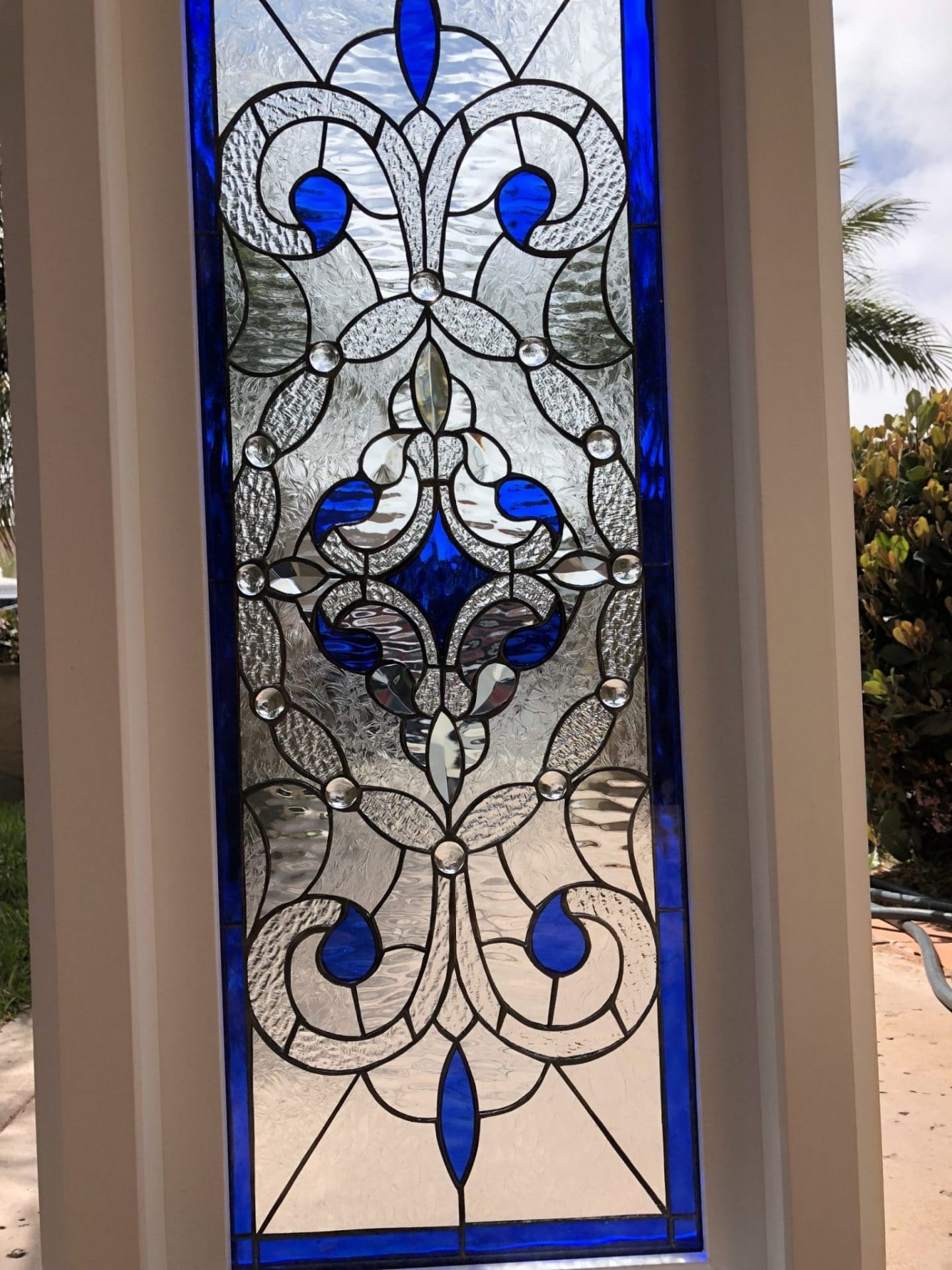This image depicts a stained glass window with a vibrant dark blue design interspersed with clear glass panels and accentuated by black framing that outlines the decorative curves, circles, and geometric patterns. The window, framed in a white wooden trim on the sides and a beige-colored frame that might be metal or dense plastic, stands out prominently against the setting. The bottom part of the window rests on concrete, with its base barely visible and the top out of frame. In the background, a tropical scene emerges with green palm trees, smaller bushes, a visible water pipe, and a bright blue sky with white clouds, suggesting the photo was taken during daylight. The lush greenery and clear sky contribute to the tropical ambience of the scene.